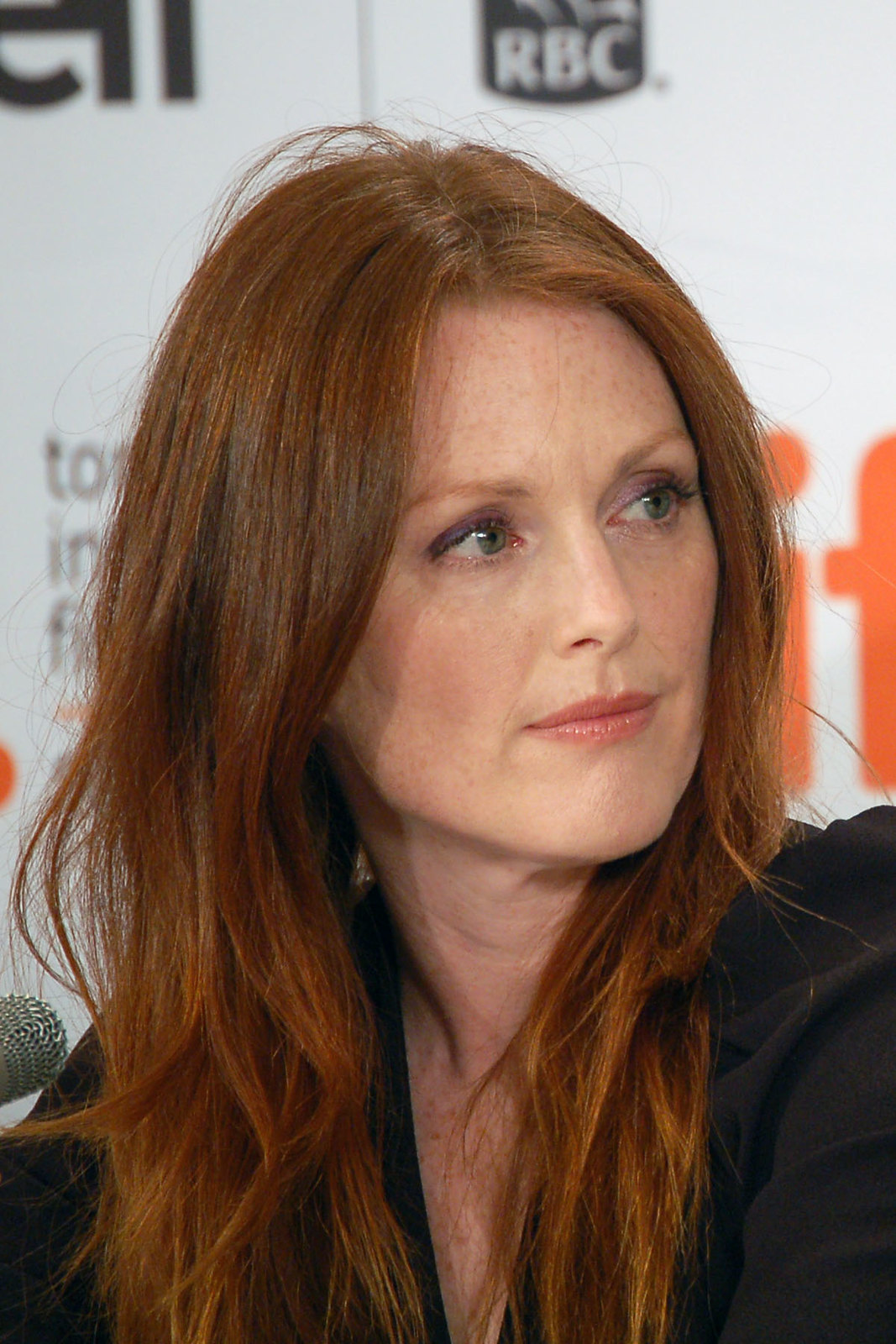The image captures actress Julianne Moore with her distinct long, amber-red hair cascading down. Her green eyes, highlighted by purple eye makeup and red lipstick, shine against her fair, freckled complexion. She is dressed in a dark-colored top with a V-neck, revealing freckles on her chest. Julianne is gazing attentively to her left, her face slightly turned. A silver-colored microphone tip is visible on the left side of the frame. The background features an out-of-focus backdrop typical of celebrity interviews at festivals, adorned with scattered, partially discernible letters, including "E," "N," "T-O," "I," "F," "R-B-C," and some orange lettering.